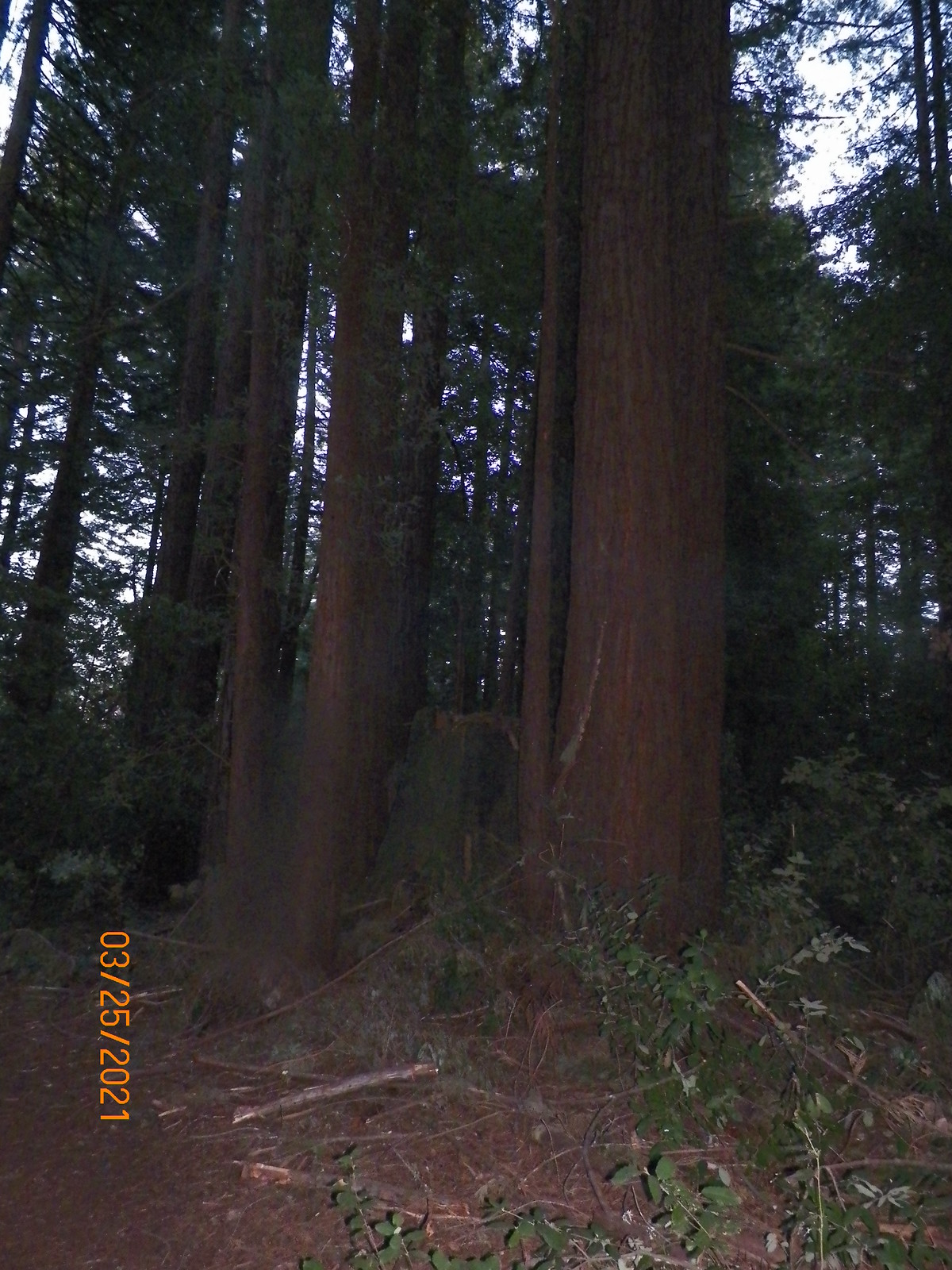The image captures a dense forest dominated by towering giant redwoods, characterized by their massive, straight trunks and reddish-brown bark. The photograph, taken almost at night or near sunset, features a shadowy ambiance with minimal light filtering through the trees. A faint flash reflection is visible on the ground in the foreground. The layout is primarily vertical, emphasizing the impressive height of the trees, although the tops and branches are largely out of frame. One particularly large tree stands prominently towards the center-right of the image. In the background, the dark green leaves and branches create a dense canopy. On the forest floor, scattered leaves, branches, twigs, and patches of dirt are evident. A patch of overcast gray sky is visible in the upper right corner. The bottom left corner of the image has an orange watermark timestamp reading "03-25-2021," indicating the date the photograph was taken.